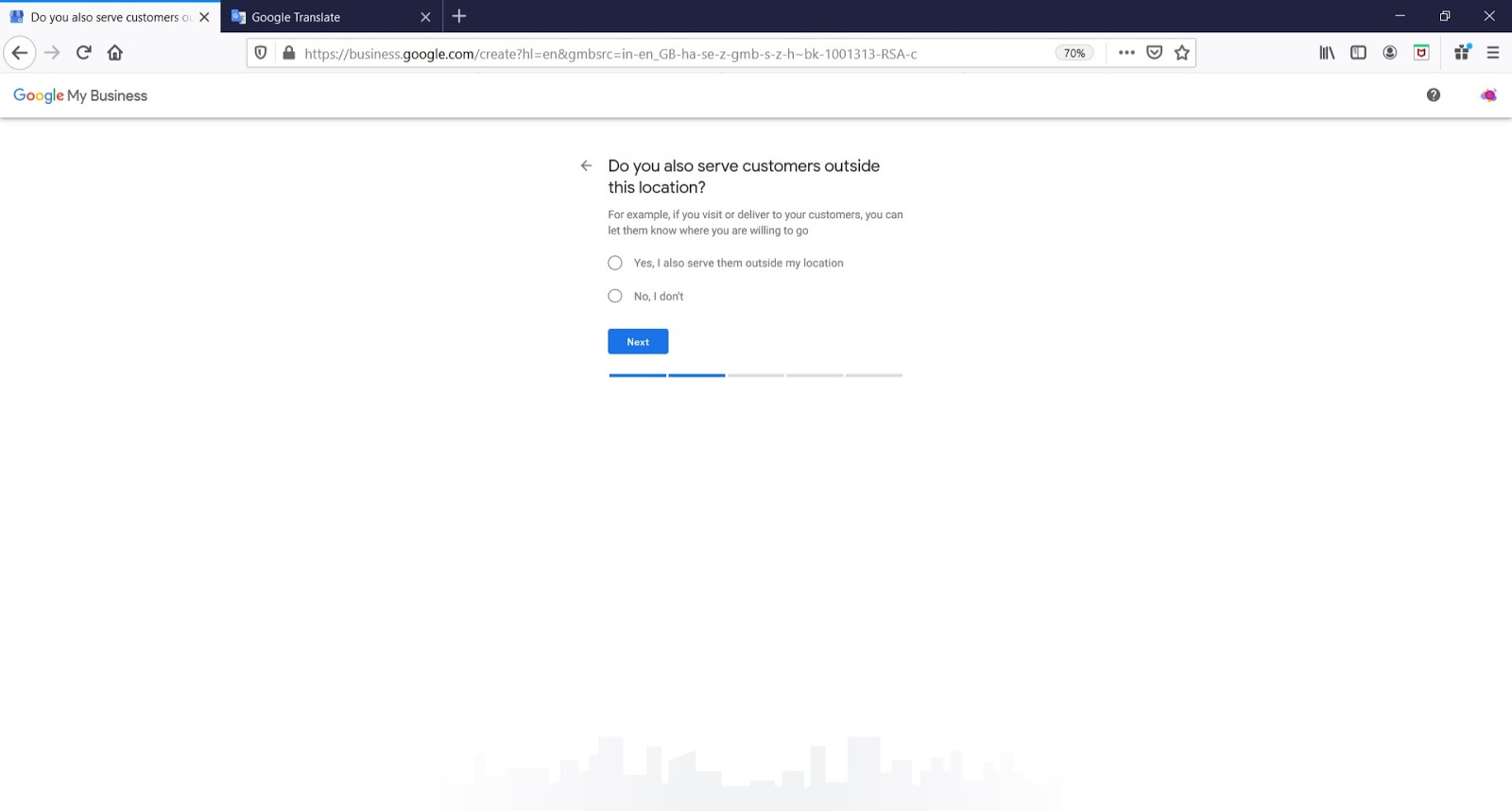In this image, we see a screenshot of a desktop or laptop computer screen displaying an open web browser window. At the top of the browser, there are two tabs visible: the first on the left reads "Do you also serve customers?" and the second one, which is not highlighted, says "Google Translate." Beneath the tabs, there's a gray bar featuring the URL and various browser tools. Below this gray bar, there's a white navigation bar with the label "Google My Business."

Dominating the center of the screen is a large white box with black text asking, "Do you also serve customers outside this location?" In smaller gray text beneath the question, it reads, "For example, if you visit or deliver to your customers, you can let them know where you are willing to go." Below this informative text, there are two radio buttons. The first radio button is accompanied by the label, "Yes, I also serve outside my location," while the second radio button, on the next line, says, "No, I don't." 

At the bottom of this white box, there's a blue rectangular button with "Next" written on it in white text. Below this section, there are clickable tabs that indicate the user's progress through a multi-step process. It appears that the user is currently on page 2 of 5, as indicated by two highlighted tabs, with three additional tabs remaining unhighlighted.